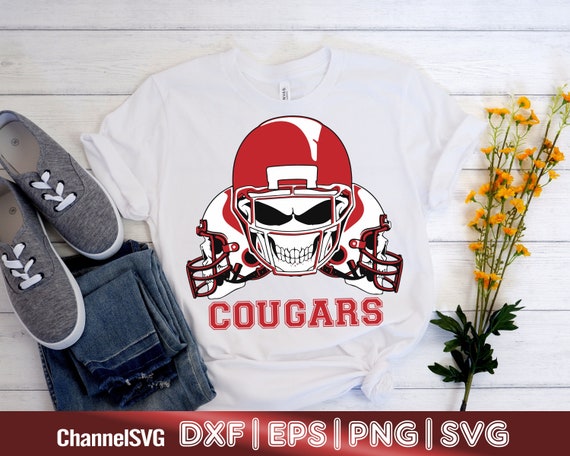The image is a professionally staged photograph likely intended for advertising, featuring various items laid out on a white wooden panel backdrop. At the focal point of the composition is a plain white, short-sleeved cotton t-shirt. The t-shirt prominently displays a silkscreen design featuring a red football helmet at the center with a menacing white skeleton face inside it, characterized by black eyes and a broad toothy grin. On either side of this central helmet image, symmetrical white helmets with red face bars also contain the same skull design. Below the helmet images, the word "Cougars" is printed in large, red, collegiate-style letters.

To the left of the t-shirt, a folded pair of blue jeans is neatly positioned next to a pair of charcoal gray low-top shoes, which feature white soles and laces. On the right side of the t-shirt, a small arrangement of yellow flowers with long green stems and some leaves is displayed. 

At the bottom of the image, a dark red horizontal banner with white text reads "Channel SVG DXF | EPS | PNG | SVG," arranged in different fonts and separated by vertical bars.